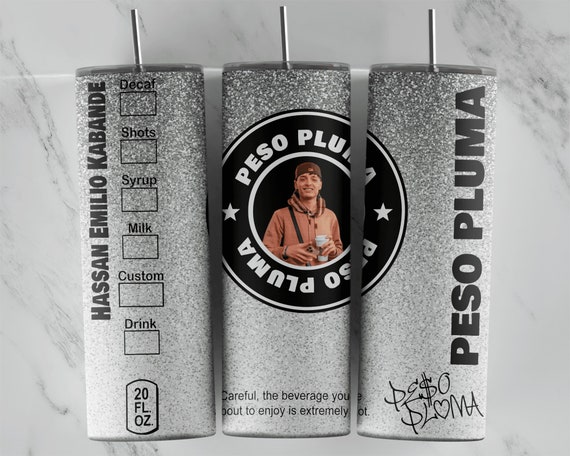In the photograph, there are three slim, cylindrical beverage cans placed in a row on a light gray tiled surface. These cans feature a gray-white speckled finish with writing and images in black and white. 

The leftmost can is vertically oriented and features text that reads "Hassan Emilio Kabandé." Below this text are rectangular boxes with labels such as "Decaf," "Shot," "Syrup," "Milk," and "Custom Drink," indicating options to customize the beverage.

The central can displays a partly visible logo that continues onto the rightmost can. The logo features a circular design with a thinner outer black line and white stars on either side. Inside the circle is a picture of a man of Hispanic appearance wearing a backwards baseball cap and a light tan hooded jacket. Around this image, the words "Peso Pluma" are written in white letters. At the bottom of this can, a warning reads, "Careful, the beverage you are about to enjoy is extremely."

The rightmost can completes the circular logo from the central can, and also features the text "Peso Pluma" written vertically, along with what appears to be a signature below.

Each can is topped with a small metallic straw, and the arrangement seems to show the different sides and details of the cans, providing a comprehensive view of their design.